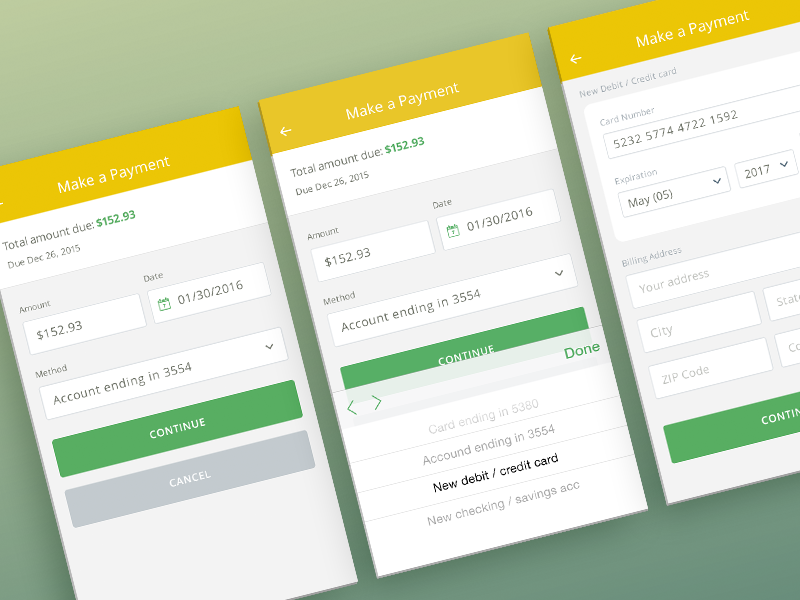The series of three images illustrates a step-by-step guide to making a payment through a mobile app. The images are set against a gradient green background and positioned diagonally from the bottom-left to the upper-right corner. Across the top of all three images is a golden bar featuring the text "Make a Payment" in bold white font, accompanied by a back arrow.

**First Image:**
- Header: "Total Amount Due"
- Amount: $152.93 in green text
- Due Date: December 26, 2015
- Input Fields:
  - Amount: $152.93 (editable)
  - Date: January 30, 2016 (editable)
  - Account: Ending in 3554 with a dropdown menu
- Buttons:
  - "Continue" in white text on a green rectangle
  - "Cancel" in gray text on a gray rectangle

**Second Image:**
- Most details from the first image are repeated.
- Changes/Additional Elements:
  - The "Cancel" button is no longer visible.
  - Two green arrows for navigation: one pointing left and another pointing right.
  - A green "Done" button.
  - A selection wheel featuring:
    - "Card Ending in 5380"
    - "Account Ending in 3554"
    - "New Debit/Credit Card" (currently selected)
    - "New Checking/Savings Account"

**Third Image:**
- Selected Payment Method: "New Debit/Credit Card"
- Input Fields:
  - Card Number: 5232577447221592
  - Expiration Date: May 2017
  - Security Code: Not visible
  - Billing Address: Options to input city, state, and zip code in editable fields
- Button: "Continue" in white text on a green rectangle

Overall, the images collectively demonstrate the process of making a payment through a mobile app, highlighting different stages and input fields required to complete the transaction.